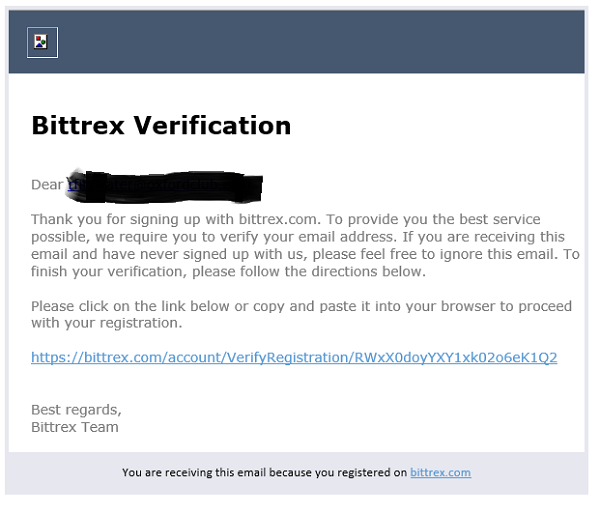The image depicts a verification page for the website Bittrex. At the top, there is a grey border beneath which lies a box with a white background containing text. The heading, in bold black letters, reads "Bittrex Verification." Below this, the text begins with "Dear," followed by a crossed-out name, indicating a redacted user identity.

The message expresses gratitude for signing up with Bittrex.com and explains the necessity of email verification to ensure the best service. It provides instructions for completing the verification process, advising users to click on a provided link or copy and paste it into their browser to proceed with registration. The URL is partially visible as "Bittrex.com/account/verify_registration/rwxx0doyxy1xk0206ek1q2." The message concludes with, "Best Regards, Bittrex Team." 

Additionally, a note informs recipients who did not sign up for the service to simply ignore the email. The structured layout and clear instructions emphasize the importance of completing the verification process to access Bittrex services.